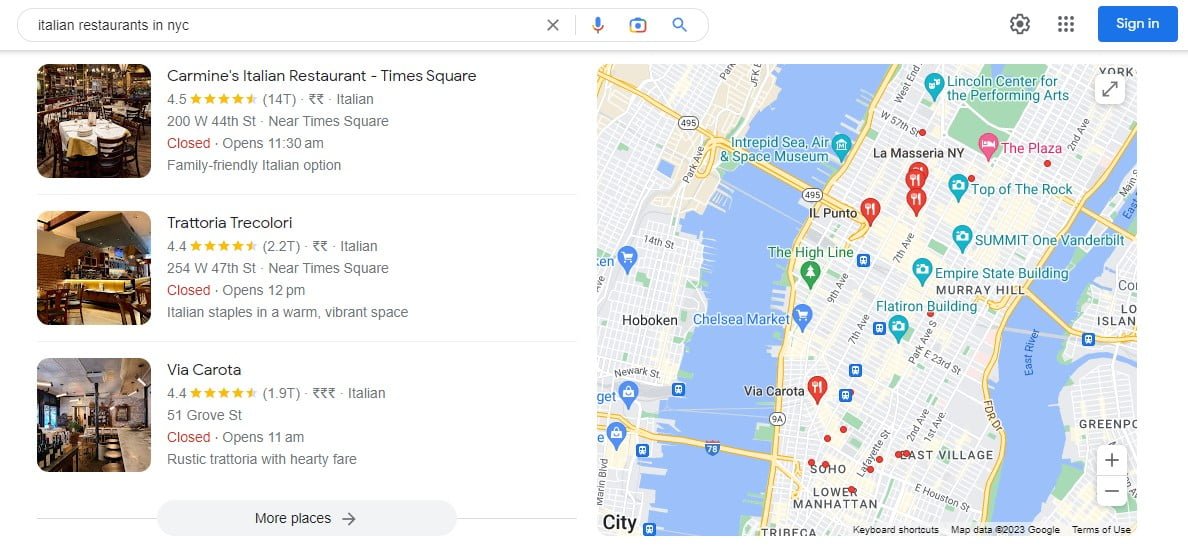The image is a screenshot resembling a Google Maps search interface. At the top, there's a prominent white search bar displaying the query, "Italian restaurants in NYC" in black text. Adjacent to the search bar on the right, several icons are visible: a microphone, a camera, a magnifying glass, a gear, and a grid of nine dots. There's also a blue "Sign in" button situated towards the far right. 

On the left side of the interface, there's a list of three Italian restaurants. The first restaurant listed is "Carmine's Italian Restaurant, Times Square," which boasts a rating of 4.5 stars. It’s described as an Italian restaurant with family-friendly options. The listing notes that it's currently closed but will reopen at 11:30 AM. The second restaurant is "Trattoria Tricolori," rated at 4.4 stars, and is known for offering Italian staples in a warm, vibrant atmosphere. The third listing is "Via Carota," also with a 4.4-star rating, described as a rustic trattoria providing hearty fare. Below these listings, there's an option to view more places.

To the right of the listings, a map of the NYC area is displayed. The map features various markers: red markers indicating restaurant locations, blue markers with camera icons, and others with cart icons. Yellow roads crisscross the map, and blue regions depict bodies of water, likely representing the ocean.